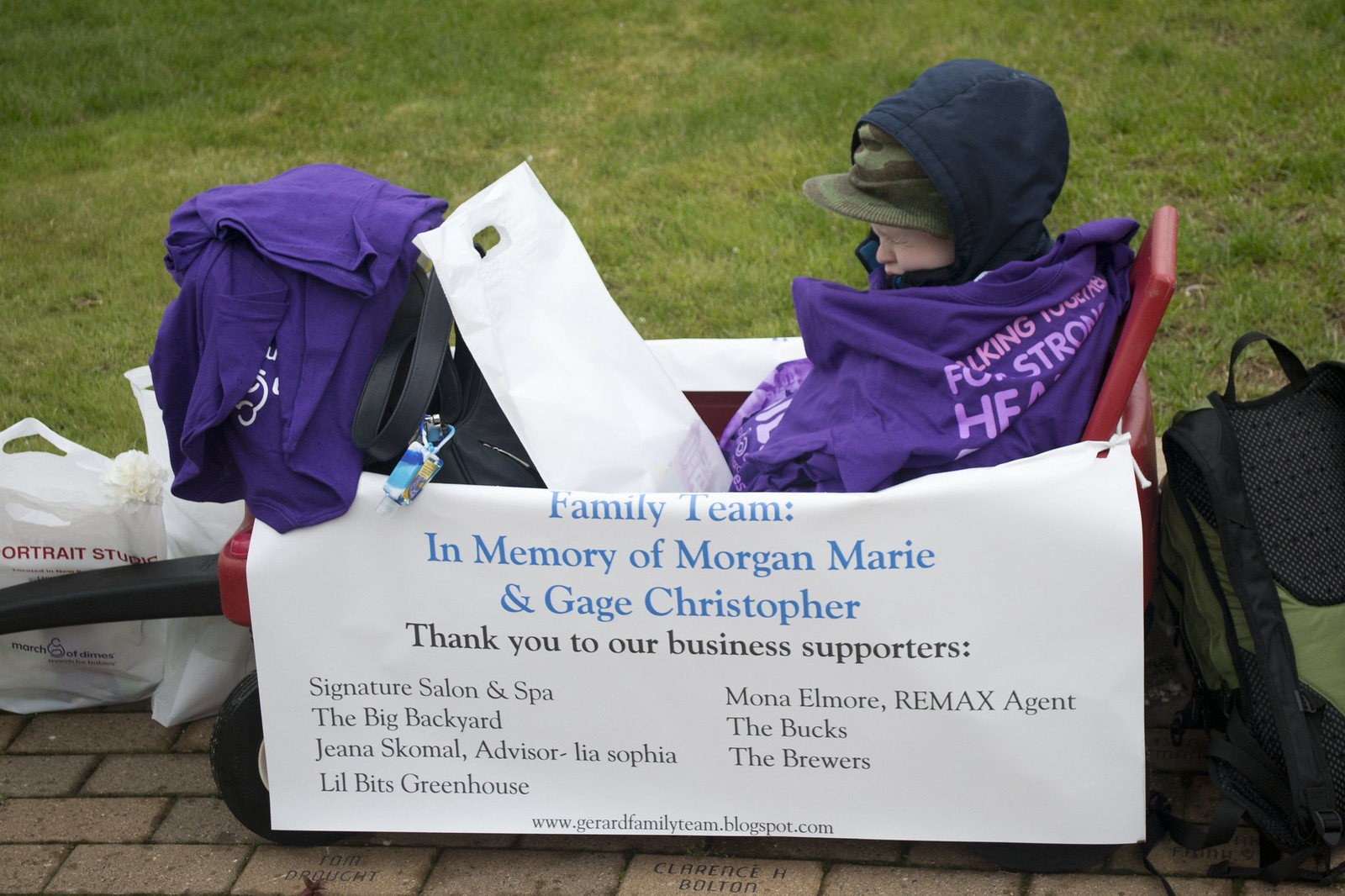In the photograph, a young child sits cozily in a red plastic wagon adorned with four black tires featuring yellow rims. The child is bundled up, wearing a purple jacket over a blue hoodie, with the hoodie pulled up over a camouflage-patterned bucket hat. The child seems to be asleep, with eyes gently closed, and leans back slightly against a white bag in the middle of the wagon. The wagon's side showcases a canvas banner with numerous lines of text that read, "Family Team, in memory of Morgan Marie and Gage Christopher. Thank you to our business supporters." It then lists the sponsors: Signature Salon and Spa, The Big Backyard, Giannis Scomo Advisor, Leah Sophia, Lil Bits Greenhouse, Mona Elmore Remax Agent, The Bucks, The Brewers, and the URL www.gerardfamilyteam.blogspot.com. In the background, lush grass can be seen, and the wagon rests on a red brick sidewalk. Also visible in the wagon are some other purple items that appear to be t-shirts.